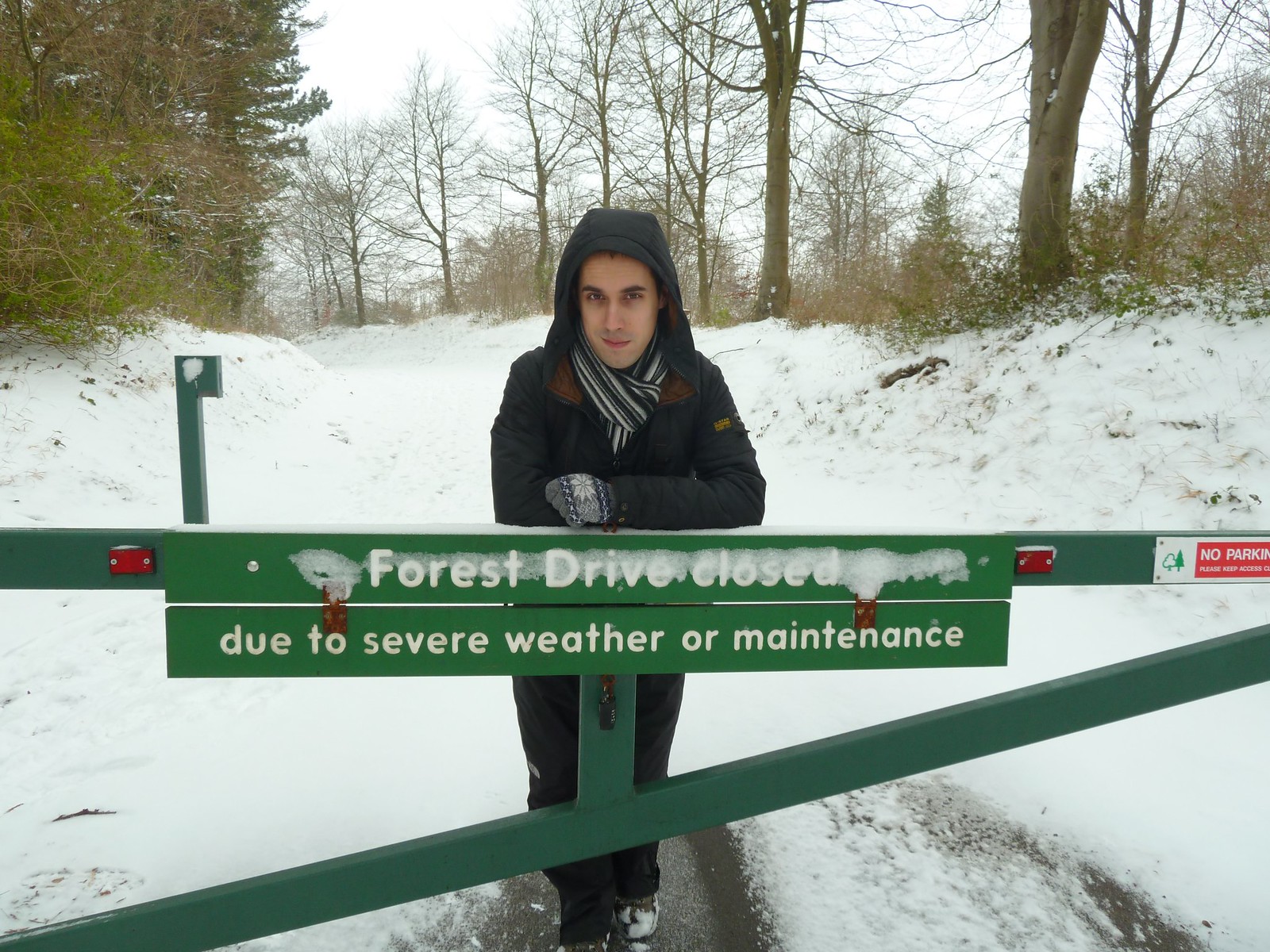In this full-color photograph, a man is standing amid a snow-covered landscape during winter. He is positioned just inside a green gate, adorned with a sign that reads, "Forest Drive Closed Due to Severe Weather or Maintenance." The sign, featuring white letters on a green background, is prominently displayed. He is a Caucasian male, likely in his mid to late twenties, dressed warmly in a blue jacket with the hood up, grey gloves, and a striped scarf. His gaze is directed at the camera, which is positioned outside the gate, and he appears to have a slight smirk on his face. The surrounding scene includes bare trees devoid of leaves and a significant amount of snow, indicating the depth of winter. Additionally, a 'No Parking' sign is visible to the left. The overall lighting suggests it is daytime, yet overcast rather than sunny.